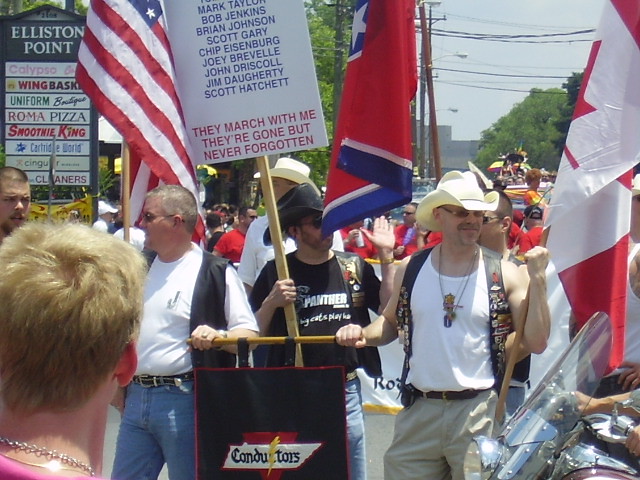The image features a large outdoor parade or rally occurring during the day on a street near a shopping area named "Elliston Point," with visible business signs for establishments such as Wing Basket, Uniform Boutique, Roma Pizza, and Smoothie King. The sky above is notably gray. The crowd consists of numerous people, some holding up flags including an American flag, a Confederate flag, and a Canadian flag. Central to the image are three white men in cowboy hats; one is waving, another raises a fist, and the third, dressed in black, stands behind a podium. This man in black holds a sign listing names: Mark Taylor, Bob Jenkins, Brian Johnson, Scott Gary, Chip Ellisonberg, Joey Breville, John Driscoll, Jim Daughtry, and Scott Hatchett, with the inscription, "They March With Me, They're Gone But Never Forgotten." Below this text, a sign on the podium reads "CONDUCTORS", with a lightning bolt symbol replacing the "C". There is a motorcycle in the lower left corner, and different clusters of people, including a group wearing matching shirts, surround the key figures. Another man in a vest converses with someone to his left, adding to the busy and somewhat somber atmosphere.